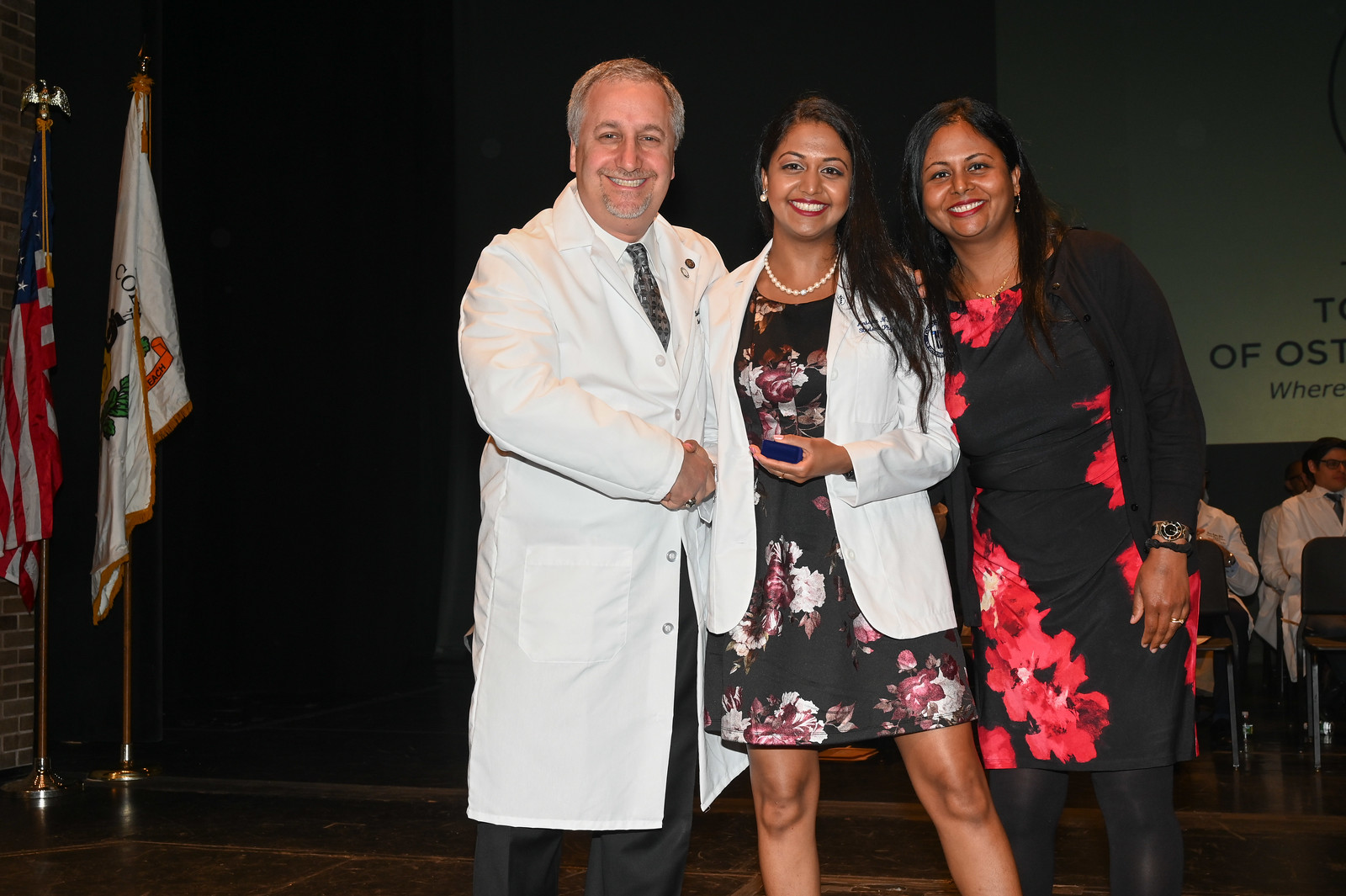The image depicts a lively and celebratory scene at an award or graduation ceremony. In the center of the photograph, three people—two women and a man—are standing close together, smiling warmly at the camera. The man, who has grayish-white hair and light skin, is wearing a white doctor’s coat, a white shirt, and a gray or blue necktie. He has a bit of gray facial hair and is shaking hands with the woman standing next to him.

This woman, who appears to be either Asian or Indian, is wearing a black dress adorned with pink and white floral patterns, complemented by a white blazer and a pearl necklace. She has long, straight, dark hair and is holding something blue in her hand, likely an award or certificate. Her earrings add a touch of elegance.

Next to her is another woman, who may be her mother, sharing a similar appearance with long, dark hair. She is clad in a black dress with floral designs and black tights, also smiling at the camera. Both women have darker skin complexions.

To the left of the trio, two flags stand tall on floor poles: one is the American flag, and the other is a white flag with some orange and green details. In the background, a few people in white doctor’s coats are seated, suggesting they are part of the same ceremony. The setting is well-lit with natural light, enhancing the vividness of the colors in the photograph.